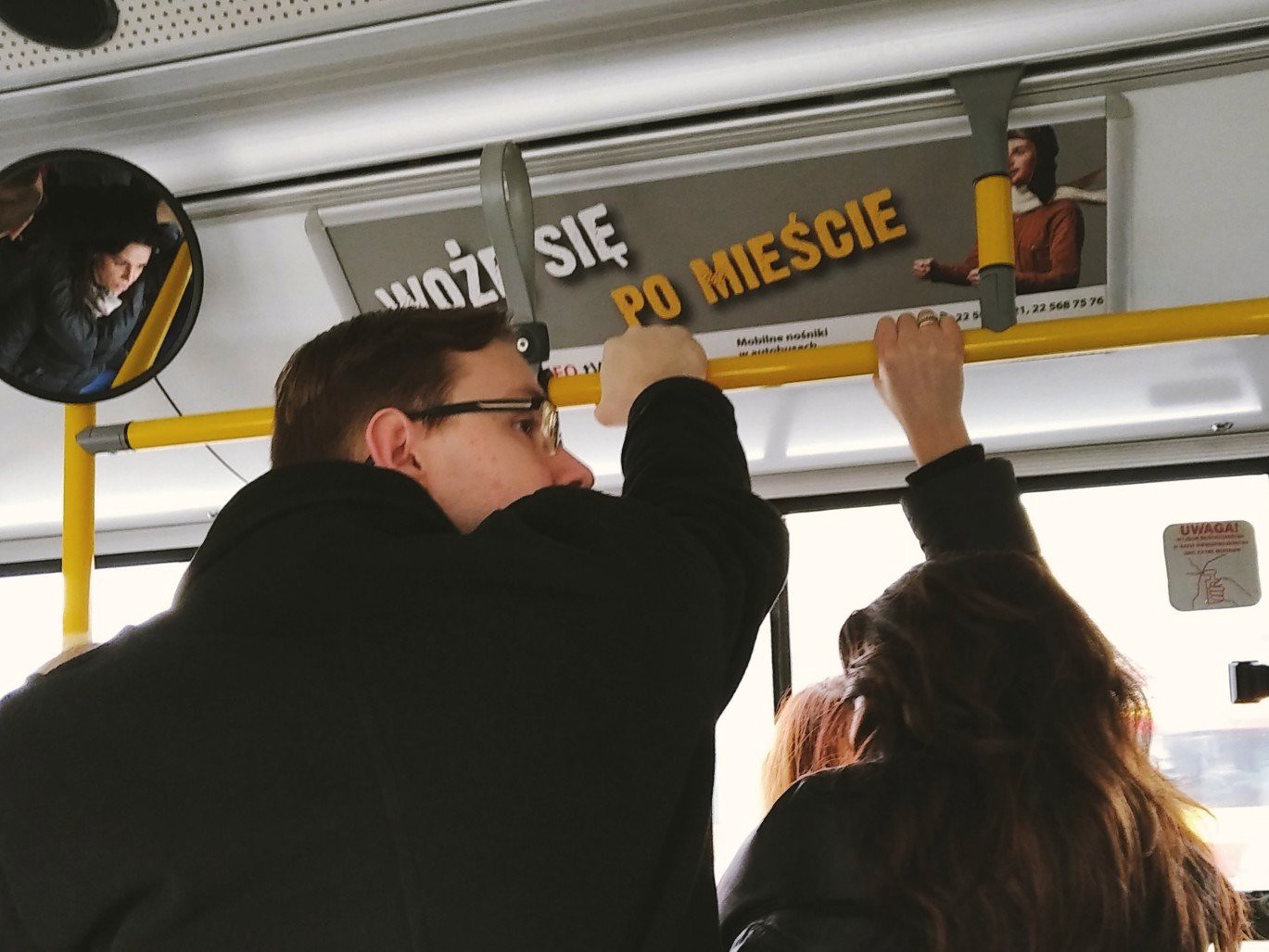This detailed photo captures a scene inside a bus. At the forefront are two individuals standing and holding onto a yellow rail that extends from the bus's roof. The person on the left is a man with short brown hair, wearing glasses with black rims, and dressed in a long-sleeved black coat. He is slightly taller and presents a side profile to the camera. The individual on the right is a shorter woman with long wavy brown hair, also dressed in a black coat. Her head reaches around his shoulder level. 

Above them, a circular mirror reflects the face of the bus driver, a woman with light skin and black hair, wearing a black coat. The window in front is brightly illuminated, making the outside view almost invisible due to the intense light. Overhead, there's an advertisement in a foreign language, featuring a mixture of white and yellow text and an image of a person in an antique-style outfit, complete with a leather pilot helmet. The partial and blocked out text includes fragments such as "W-O-Z," "S-I-E," and "M-I-E-S-C-I-E."